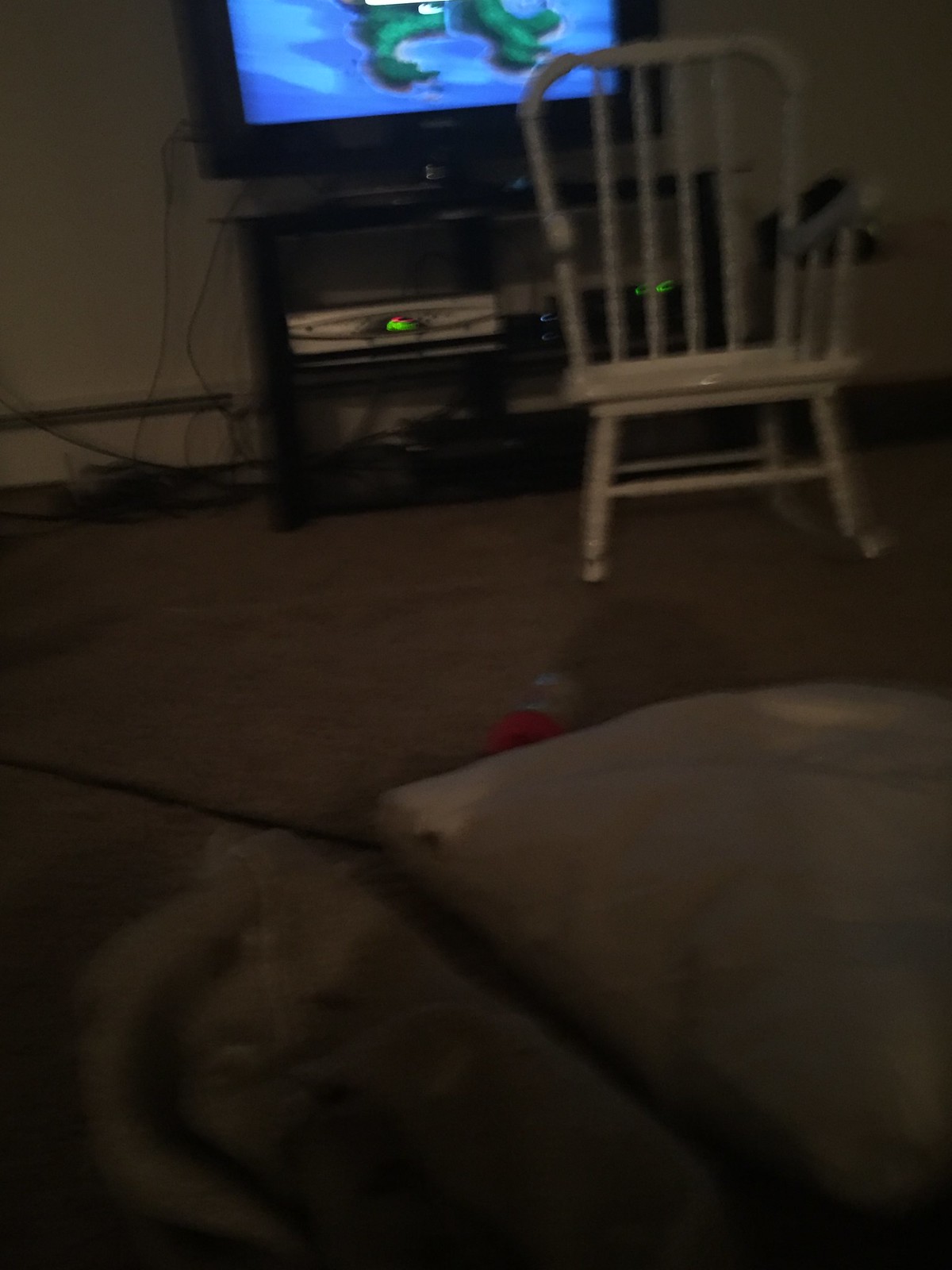The image, slightly blurry and taken from a low perspective, appears to be of a cozy room within a house or apartment, either a living room or bedroom. The viewpoint, which seems to be from someone laying on brown-cushioned furniture, captures several key elements of the space. Dominating the foreground is a dark-colored carpet and a hint of a gray pillow. Positioned centrally and slightly to the right is a white, wooden rocking chair with curved rockers, cylindrical back poles, and armrests, positioned in front of a TV on a short entertainment center. The TV, black and turned on, displays a partly visible blue and green screen, possibly an animated show. The wall behind the TV is plain white or off-white, contributing to the room's simple decor. The entertainment center also holds various electronic devices, distinguished by green lights but indiscernible due to the image's blurriness. The vertical, skewed angle of the photo adds to the room’s intimate, lived-in feel.